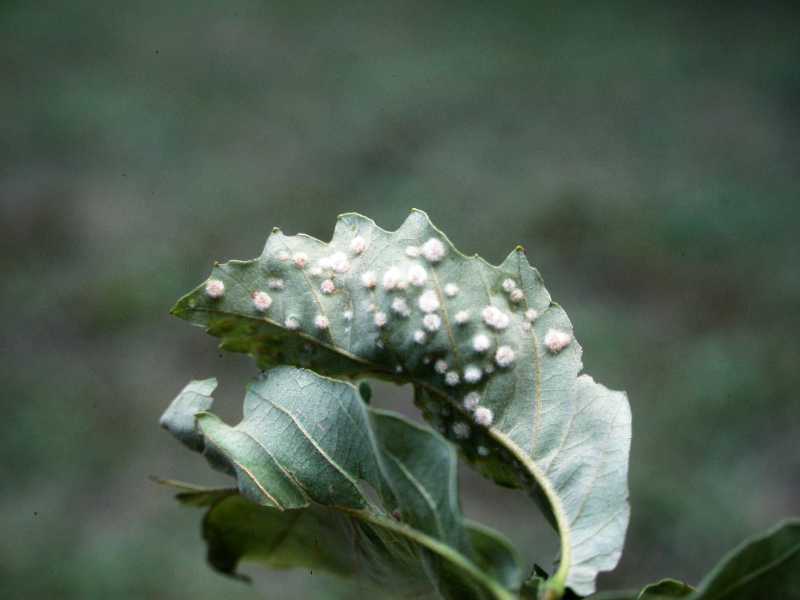This detailed photograph showcases an extreme close-up of two light green leaves against a deeply blurred green and dark background. The primary leaf, viewed from its underside, appears slightly curved and somewhat dry, displaying a multitude of growths. These growths, likely indicators of disease or insect activity, resemble white, puffy cotton balls or corpuscles, with some larger and others smaller. Covering about two-thirds of the leaf's surface, they sporadically dot the leaf without a discernible pattern, creating a textured landscape of fuzz-covered protrusions. In contrast, the adjacent leaf, viewed from its front, remains unscathed, adding a comparison point in this complex depiction. This image, possibly significant for those studying plant biology or horticulture, captures the afflicted leaf's struggle against what appears to be a parasitic or fungal invasion, highlighting the stark contrasts between health and disease in plant life.